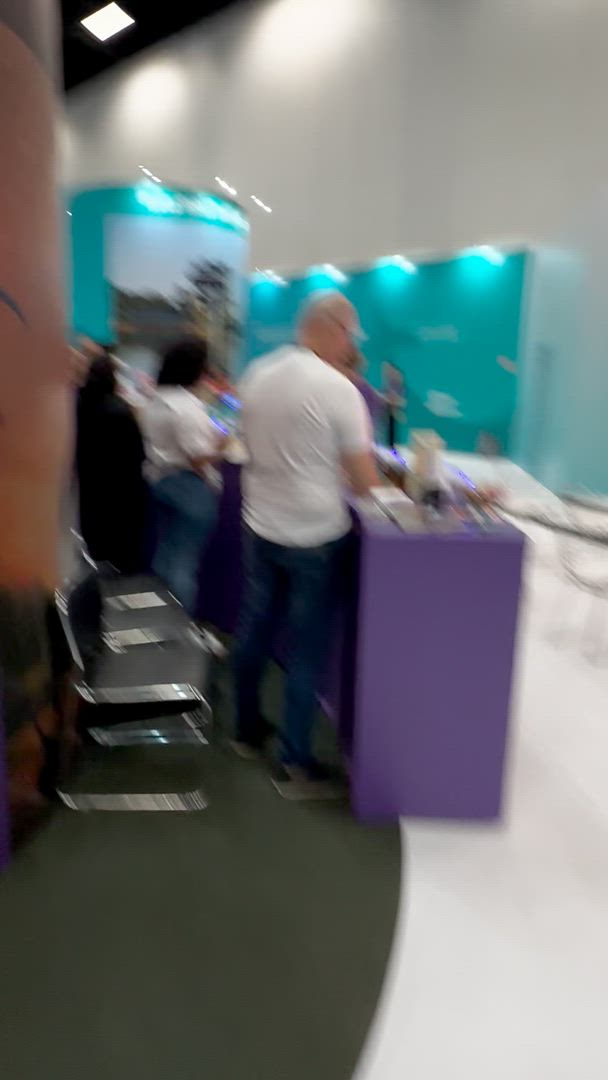This image, though very blurry, depicts a scene at a trade show or fair. In the foreground, two individuals stand behind a waist-level, purple counter cluttered with various items, possibly indicating products for sale or display. The man, positioned on the left, has a bald head or very short haircut, possibly wearing a small-rimmed baseball cap, glasses, a white t-shirt, blue jeans, and black tennis shoes with gray accents. To his left, a woman with shoulder-length dark hair wears a white short-sleeve blouse and blue jeans. The counter they man is set against a backdrop of intriguing visual elements.

The background reveals two black office chairs with silver trimming, likely holding receipts or tags. The wall behind them features a combination of dark brown wood and black sections, with lights highlighting a blue panel near the top. The floor, predominantly white tile, has green elements and a black runner. Intriguingly, the setting shows hints of a curved design space, possibly a booth, with additional background items, including what may appear as teal display structures or storage areas akin to porta-potties.

Decorative ceiling lights and shelves are vaguely discernible on the back wall, adding to the exhibit-like ambiance of the image.